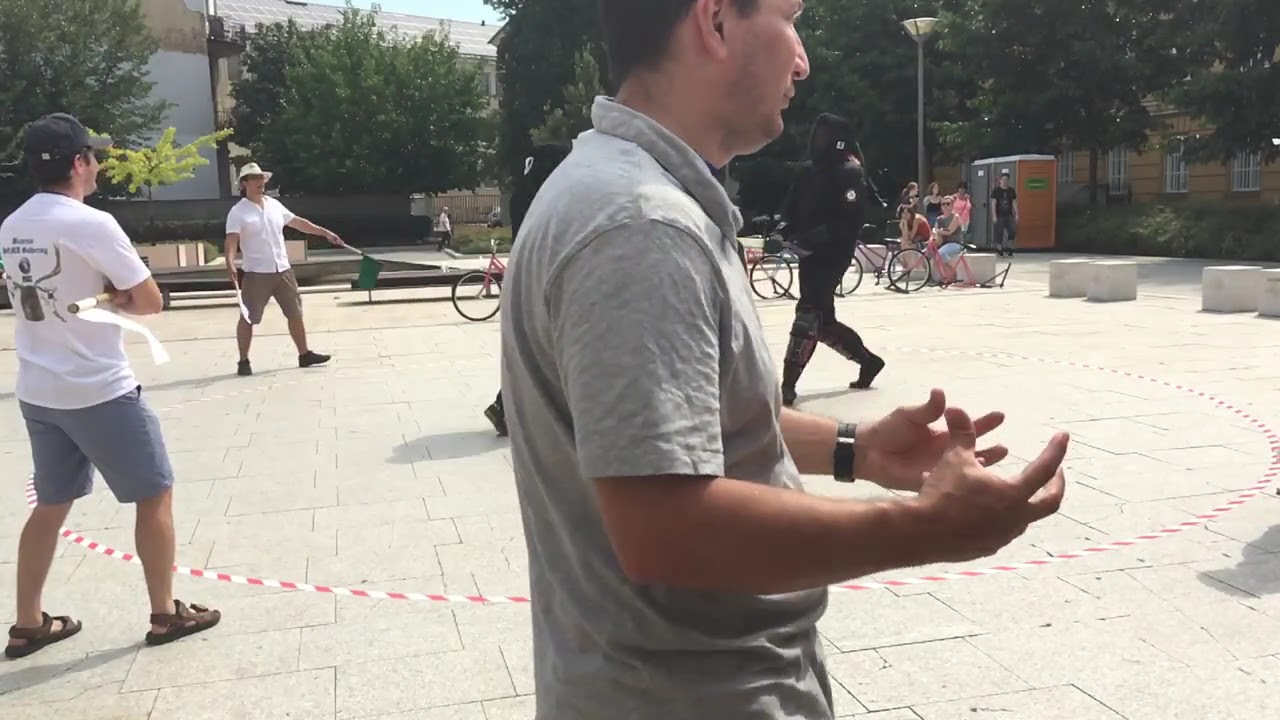The image depicts a lively outdoor scene in what appears to be a suburban park, featuring a hard cement ground with flat stone tiles arranged in square and rectangular shapes. At the center of the scene, a thin, red and white striped ring forms a circle, suggesting the setup for a possible combat competition. A young man in the foreground, dressed in a light gray shirt with a watch, holds his hands awkwardly at a 90-degree angle, as if pinching his fingers together. He has short brown hair and is looking to the right. To his left stands another man in a white T-shirt, light gray shorts, and brown flip flops. In the background and within the ring, a figure dressed in black, including a face mask helmet, stands poised, suggesting he might be participating in the aforementioned combat activity. A referee holding a white and green flag is visible on the left side of the image, overseeing the event. Additional spectators, some with bicycles, can be seen gathered around, along with a few trees and buildings that add to the suburban ambiance.